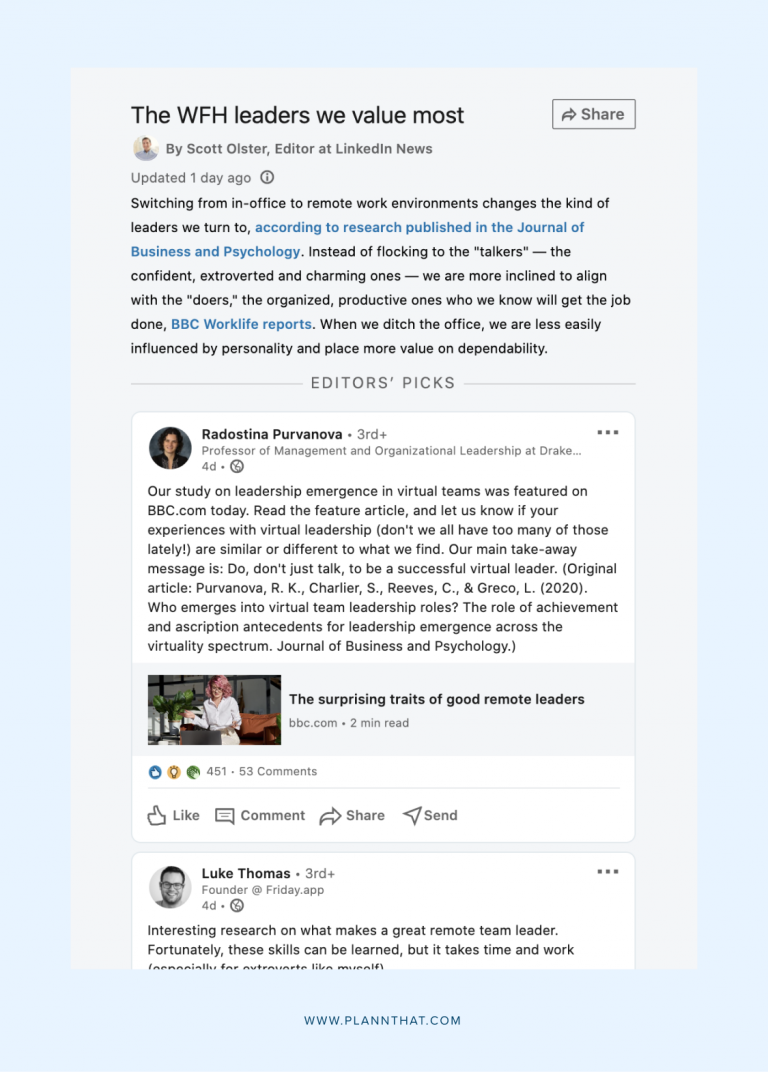Here's a detailed and cleaned-up caption for the image:

---

This is a screenshot of a page from PlanThat.com, identified by the blue-colored bottom border. The page has a light blue border and features what appears to be a blog post with embedded social media screenshots. Title at the top reads, "The WFH Leaders We Value Most," in black text. To the right, there's a gray share button with a darker gray shade that includes a share arrow and the text "Share" next to it.

Below the title, there is a small round icon of a male's portrait. Next to it, it reads, "By Scott Ulster, Editor at LinkedIn News," followed by "Updated one day ago" and an information icon. The main content highlights a shift in leadership preference from "talkers" - the confident, extroverted, and charming personalities - to "doers" - the organized and productive individuals - as shown by research published in the Journal of Business and Psychology and reported by BBC Worklife.

Following the main article, there's a section titled "Editor's Picks," separated by line breaks. This section includes a social media post that seems to be from Facebook or LinkedIn. The post is by "Radocina Pervonova," a third connection, featuring a round headshot icon and her title "Professor of Management and Organizational Leadership at Drake...". The post was published four days ago, noted by a small world icon indicating it is public. Pervonova shared details about their study on leadership emergence in virtual teams featured on BBC.com, encouraging readers to compare their experiences with virtual leadership.

Furthermore, Pervonova's post emphasizes that to be successful virtual leaders, individuals need to act rather than just talk. The original article citation follows, listing the authors and title: "Who Emerges into Virtual Team Leadership Roles: The Role of Achievement and Ascription Antecedents for Leadership Emergence across the Virtuality Spectrum," published in the Journal of Business and Psychology.

Underneath Pervonova's post, there's a banner image of a professional-looking woman. The text alongside reads, "The Surprising Traits of Good Remote Leaders" from BBC.com with a note of a "two-minute read." There are icons showing 451 reactions and 53 comments, including options to like, comment, share, or send.

Another post in the feed from Luke Thomas features a black and white headshot. Thomas, identified as the founder of Friday.app, shared his thoughts on research about great remote team leadership, noting these skills can be learned but require effort, especially for extroverts like himself. However, the post is cut off and the remainder is not visible.

---

This caption provides a clear and detailed description of the image content.